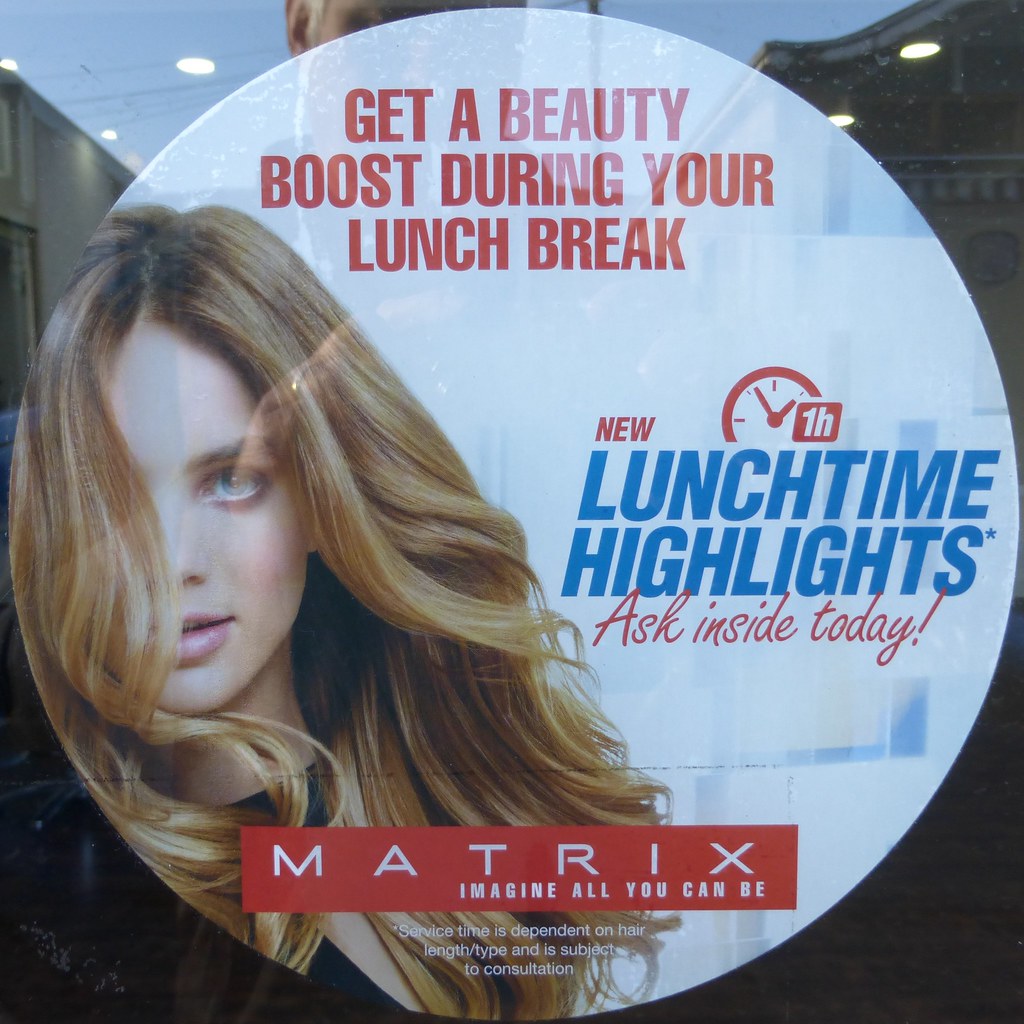This color photograph, taken outside during the day, features a close-up of a circular advertisement on the window of a hair or beauty salon. The advertisement prominently displays a young adult woman with long blonde hair cascading down her left side, partially obscuring her eye, nose, and mouth. Her visible eye is bright blue, and she wears pink lipstick and a black shirt. Reflections in the glass reveal buildings in the background and even the photographer. The ad invites potential customers with vibrant text: "Get a Beauty Boost During Your Lunch Break" in red capital letters at the top, and "New One-Hour Lunchtime Highlights" in blue on the right side. At the bottom, within a red rectangle, it says, "Matrix, Imagine All You Can Be" in white font.